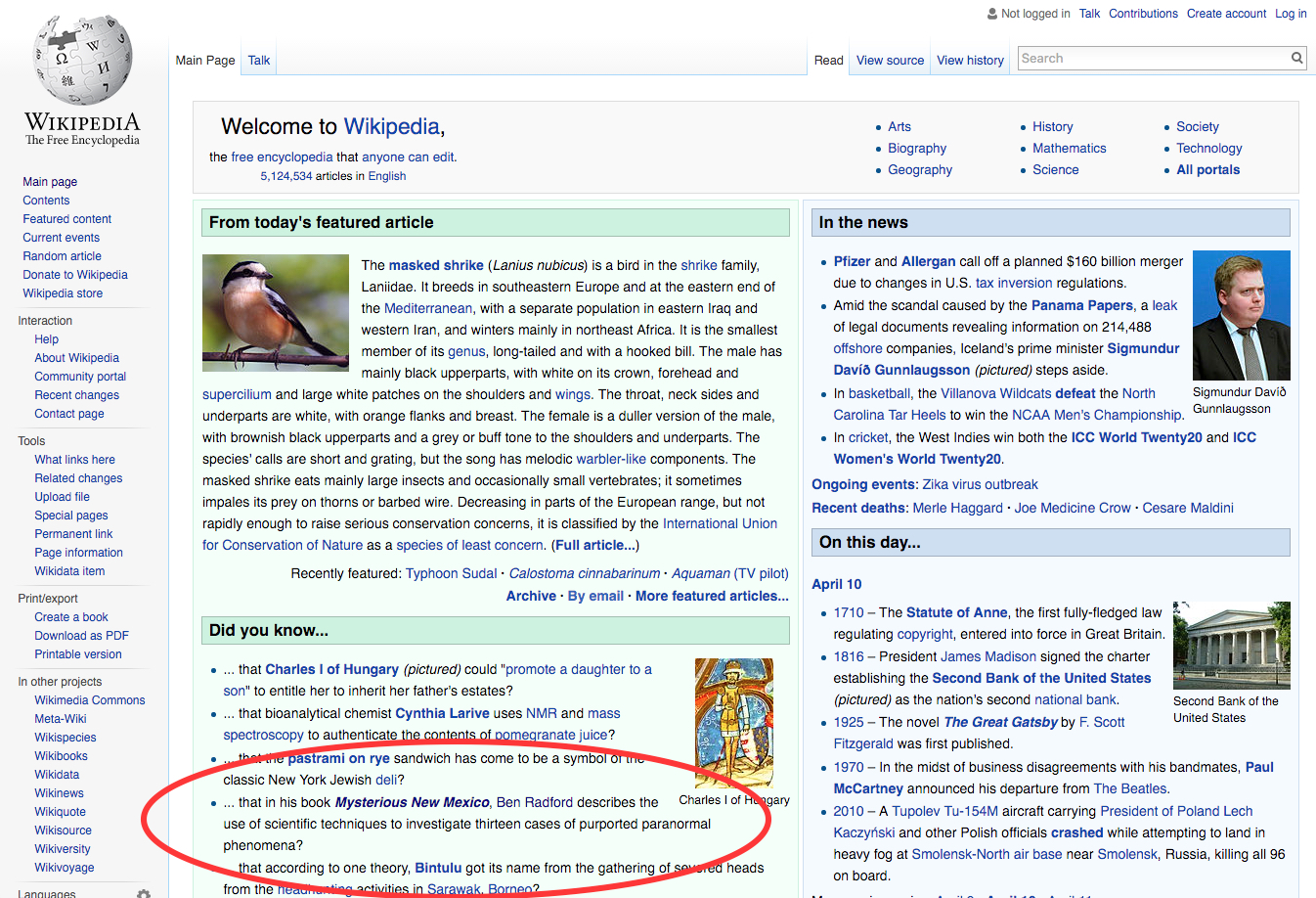This image, taken from a computer screen, showcases the main page of Wikipedia. At the top, the iconic header reads, "Welcome to Wikipedia, the free encyclopedia that anyone can edit." Beneath this headline, the page highlights that it hosts 5,124,534 articles in English. The featured content for the day is about the Masked Shrike, a bird in the shrike family. The brief description elaborates that this bird breeds in southeastern Europe and the eastern Mediterranean. Additional details and a complete article can be accessed through a provided link.

The background of this section has a light green hue. Scrolling down, there is a section titled "Did You Know," which includes four intriguing bullet points. One of these points, specifically circled in red, states: "In his book, Mysterious New Mexico, Ben Radford describes the use of scientific techniques to investigate 13 cases of purported paranormal phenomena." This circled area is highlighted by a red, oblong digital marker.

To the right, there are two columns in a bluish color labeled "In the News" and "On This Day," providing updates and historical facts respectively.